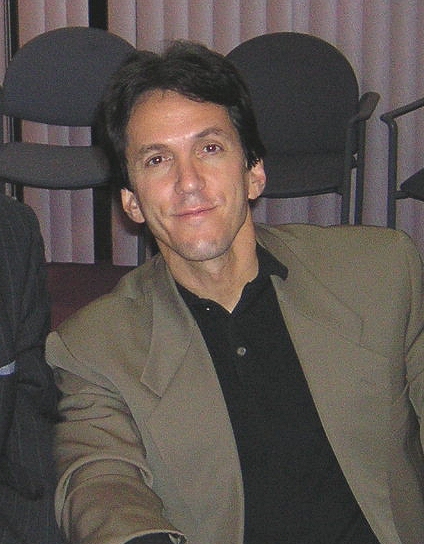This photograph features a man who appears to be an actor. He is sitting cross-legged on what looks like a stage with a backdrop of white vertical blinds and several gray office chairs, suggesting a convention or similar event setting. The man has dark, possibly Italian, features, with dark brown eyes and dark hair. He is clean-shaven and wears a light tan blazer over a black polo shirt with the top button undone. To his right, another man stands wearing a gray pinstripe coat. The stage's flooring is carpeted in gray. The actor's face seems familiar, though his name remains unrecognized. The overall composition, with its seating arrangement and backdrop, suggests a formal or semi-formal event.